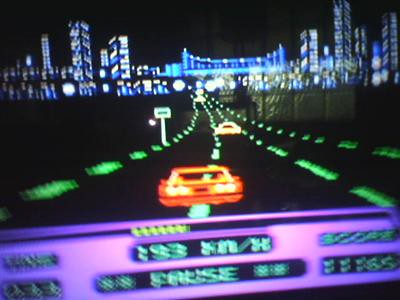This image captures a somewhat blurry screenshot of a video game displayed on a TV or computer monitor. The game depicts a nighttime highway scene with a distinct third-person viewpoint of an orange car driving amidst a few others. Despite the blur, it's evident that the image's aspect ratio is a bit wider than it is tall by approximately 20%. The road in the game is completely black, divided into four lanes by bright lime green dashed lines, and the orange car, slightly off-center between the first and second lanes, encounters a white car directly ahead. In the distance, a detailed cityscape emerges, adorned with numerous skyscrapers showing illuminated windows indicating occupied rooms. Towering above the skyline, a suspension bridge adorned with small lights is visible.

A horizontal UI bar occupies the bottom third of the screen, predominantly light purple with sections of black background inlays featuring teal or light blue text. This includes a paused status indicated by “**paused**” and a speed reading of “193 km/h.” Additional information, such as a score reading “1185,” is also spotted in the bar. The in-game display includes other cars: a red car in one of the middle lanes and a yellow car also ahead, reinforcing the urban race setting. The overall visual ambiance underscores the dynamic and fast-paced nature of the video game, all set against a vibrant yet dark backdrop.